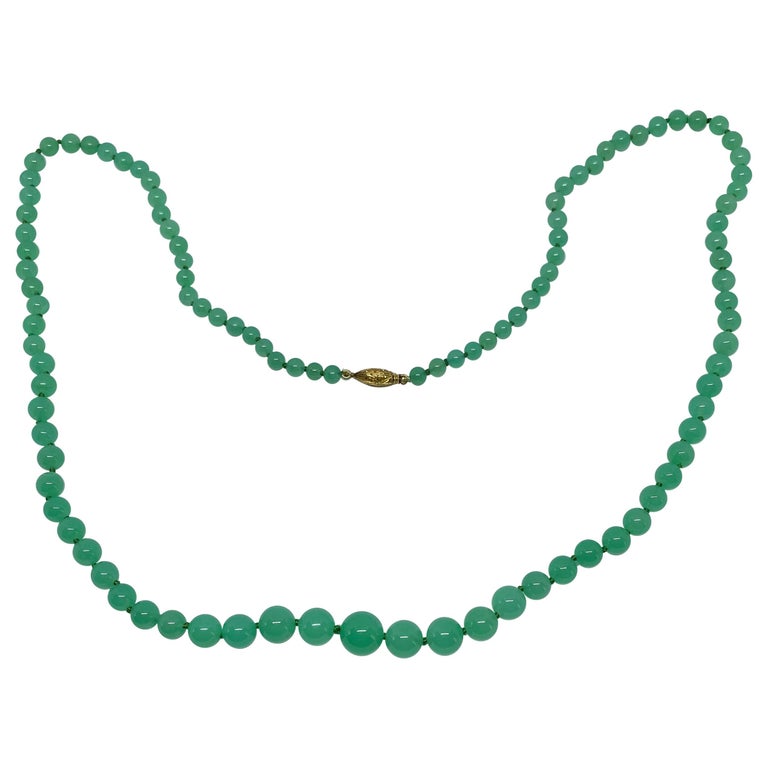This horizontal image showcases a beautifully detailed green necklace laid against a plain white background, suggesting a professional photography setting. The necklace features a string of round green beads that vary in size, starting small near the golden clasp at the top center and gradually increasing in size towards the bottom, where the largest beads are situated. The beads appear glossy, with the larger ones reflecting light as evidenced by small white spots. The necklace is arranged in a semi-circle reminiscent of a smiling mouth, extending across the surface in graceful curves and folds. The overall impression is one of simple elegance, emphasizing the natural beauty and craftsmanship of the green beads and their delicate variation in hue throughout the piece. If worn, the necklace would hang down the chest quite noticeably, an elegant accessory suitable for any occasion.